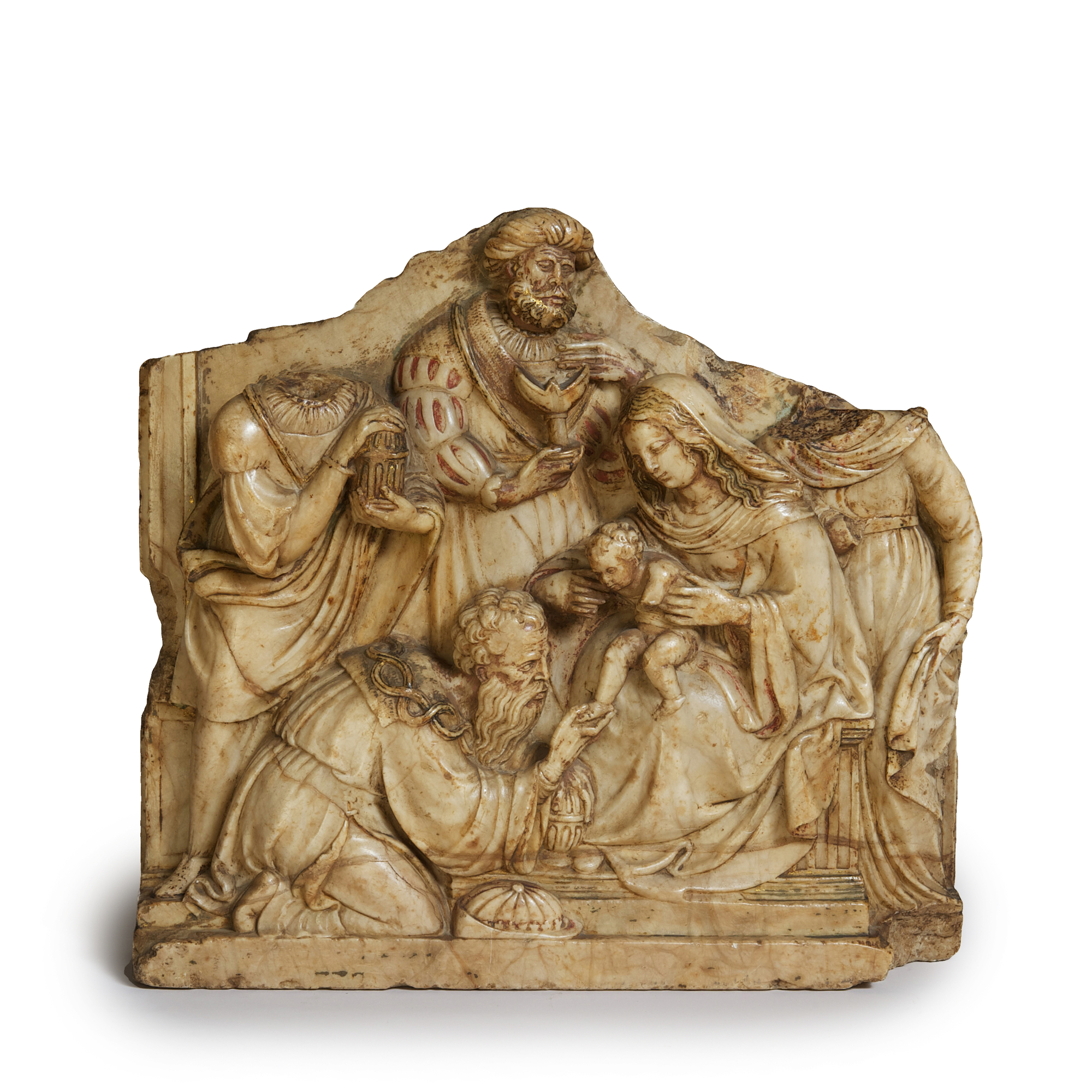The image depicts a detailed stone carving, possibly made from beige marble, showcasing a religious or historical scene. The central focus is a woman seated with a baby in her lap, intricately dressed with a veil, clearly visible strands of hair, and the baby's legs and feet. At her feet, an elder man is kneeling, washing or touching the baby's feet with a reverent expression. Surrounding this primary scene are three additional figures, most of whom are dressed in long, baggy robes typical of Renaissance or ancient times. Unfortunately, the piece is damaged, as it appears that two of these figures have missing heads, suggesting they may have broken off over time. One figure without a head holds a vase, while another man stands holding a chalice. There is also the outline of an additional person behind the woman. The entire carving is uniform in color, a shiny, intricate tan stone, highlighting the detailed craftsmanship of the period.